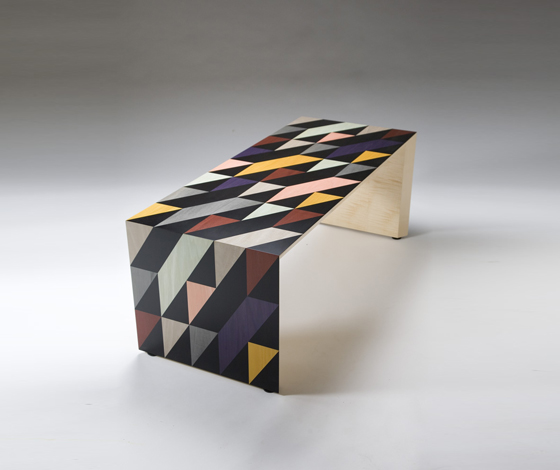The photograph captures a stylistic table placed in a large, empty room with a white floor that transitions to a darker gray towards the top of the image. The table boasts a thin surface and equally slender legs crafted from light brown wood, positioned at each corner. The most noticeable leg is located at the bottom left of the photo. The table's surface is adorned with a striking geometric pattern composed of alternating triangular shapes. These triangles present a diverse array of colors, including brown, black, gray, blue, yellow, purple, pink, and light green. Importantly, no two adjacent triangles share the same color, creating a visually compelling mosaic. The room's ample natural lighting emphasizes the clarity of the photograph, allowing every intricate detail of the table's design to stand out prominently.